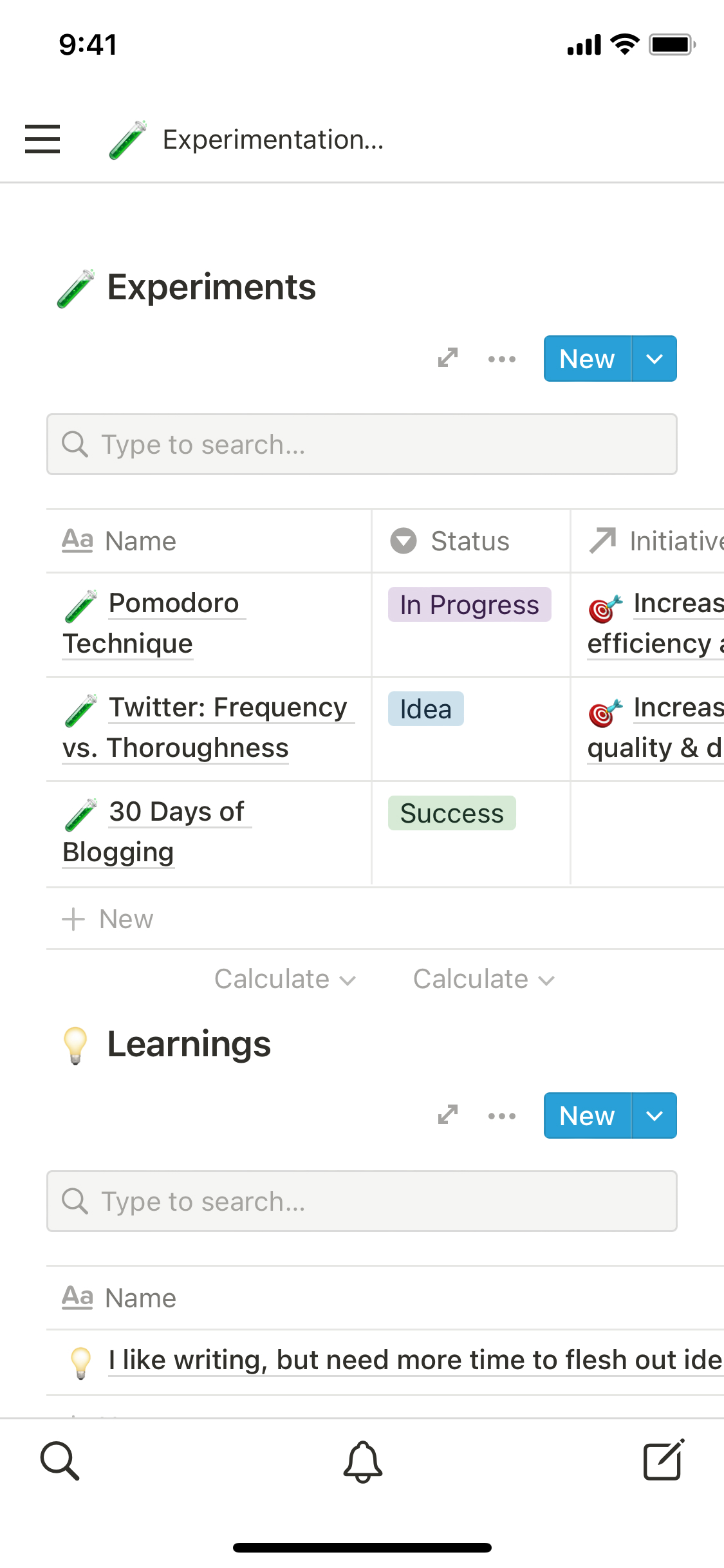A detailed cell phone screenshot displays a white background with black text at the top. The top left corner shows "9:41" while the top right depicts full service, Wi-Fi, and battery icons. Beneath this, three lines of text are shown.

In the center, there's an image of a test tube containing green liquid, labeled "Experimentation..." in grey text. Below this, a grey bar spans across the screen, repeating the test tube icon and caption "Experiments." 

In the bottom right corner, a grey arrow points diagonally, followed by three dots and a blue button with white text saying "New." Adjacent is a grey search bar with placeholder grey text reading "Type the search."

Further down, a section labeled "A" lists various statuses and initiatives. Each entry features the green-liquid test tube icon with the status marked as "Success." Initiatives like "Monto technique – in progress," "Increase effect inefficiency," "Twitter frequency vs. idea," and "30 days of blogging" are noted.

A "Plus New" button sits nearby. Centrally located are two "Calculate" options noted as drop-down menus, alongside an icon of a light bulb above the word "Learning" in black text. The grey arrow and blue button repeat here, next to another search bar.

Towards the bottom, a grey label "Name" and black text declaring "I like writing but need more time to flesh out IDE" are visible. The screen concludes with a row of icons: a magnifying glass, a bell, and a piece of paper with a pencil located in the bottom right corner.